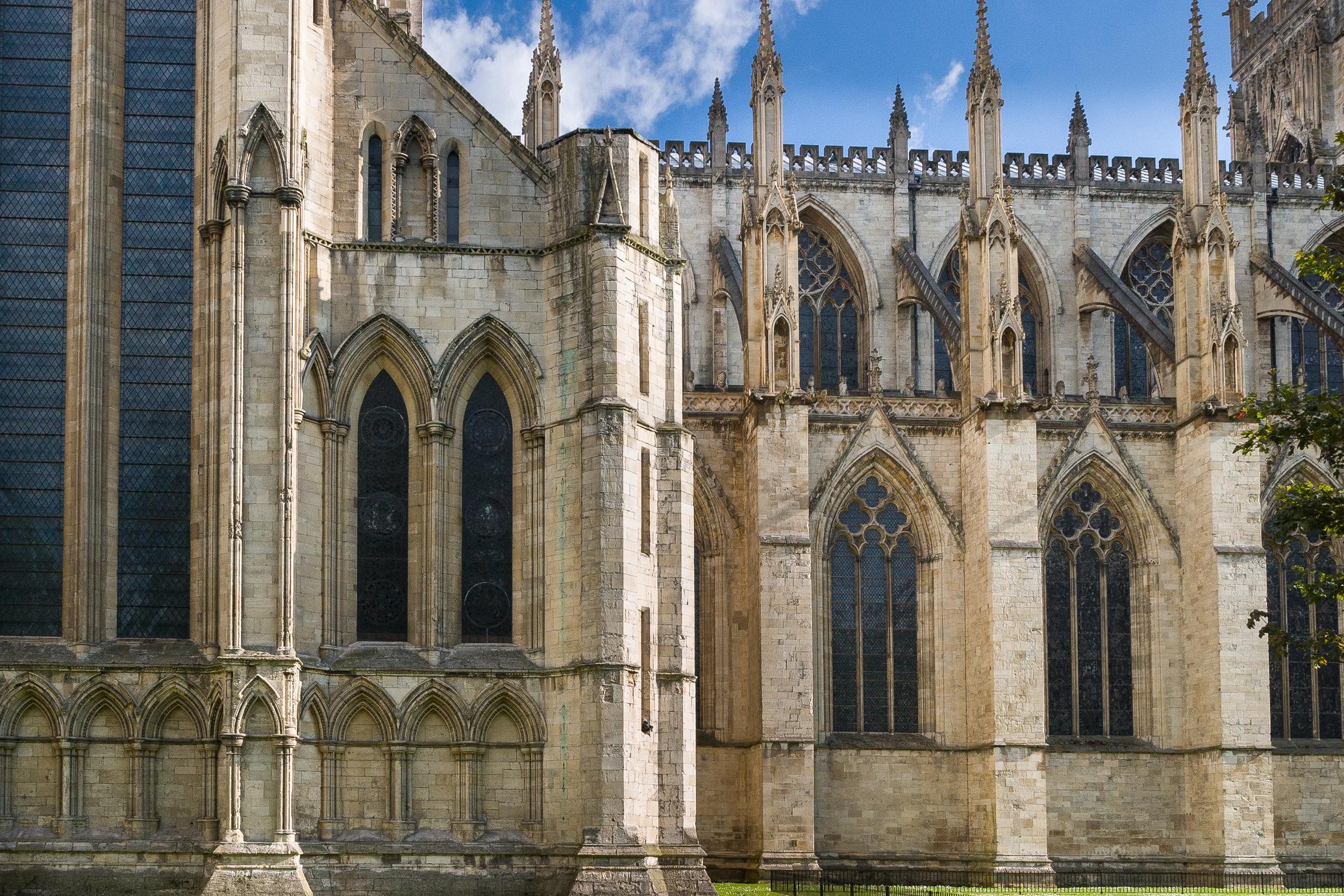This image captures the exterior of what appears to be the Notre Dame Cathedral in Paris, showcasing its grand and intricate gothic architecture. Dominating the view is a large, tall, and ornate tower on the left, possibly reaching up to four stories high. The cathedral, constructed from white or light tan stone, features several pointed turrets and flying buttresses that add to its medieval charm. The windows, especially striking, are long and arched, with ornate cross and clover-like designs. Some windows extend vertically in two- or three-story segments and are framed by square pillars that run the full height of the building. The stone surfaces of the structure are adorned with numerous spires and detailed decorative elements. The sky above is a clear blue with white clouds, emphasizing the height and elegance of the building. On the right side, a touch of greenery with trees bearing lush green leaves provides a natural contrast to the architectural splendor of the cathedral.